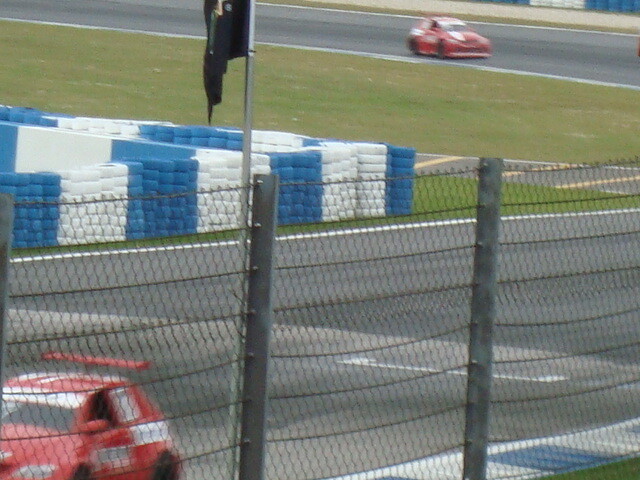The blurry photograph captures the dynamic scene of a racetrack, dominated by the presence of two identical red race cars adorned with white livery, hurtling down the grey tarmac at such speeds that their numbers and lettering are rendered illegible. The track itself is bordered by solid white lines, distinguishing it from the well-maintained grassy infield where stacks of tires, painted blue and white, serve as barriers and safety features. The tires are piled 6 to 8 high and 4 to 6 across, adding a colorful yet functional visual element. An 8-foot tall chain link fence supported by multiple posts spans the front of the image, with a black flag fluttering on a silver flagpole situated towards the left-hand side. The fence, along with the tires, signifies the protective measures in place. In the lower-left corner, one of the red race cars can be seen more distinctly, while the other flashes by in the upper left, emphasizing the thrilling, speedy nature of the event.